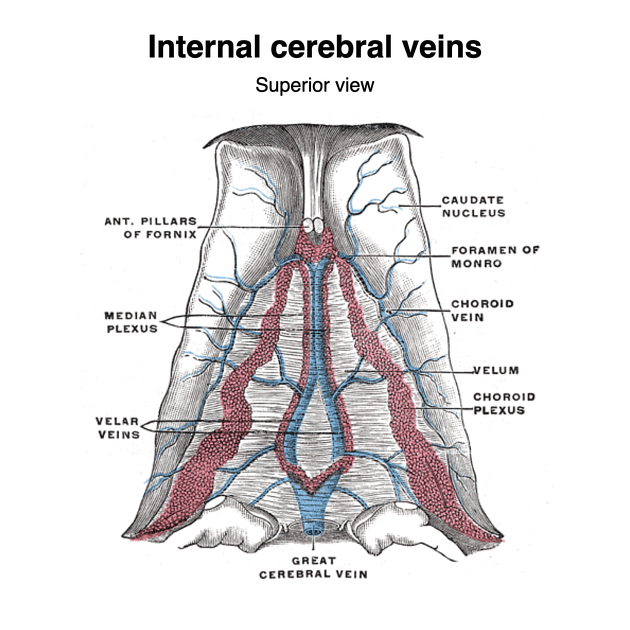The image is a detailed medical drawing titled "Internal Cerebral Veins - Superior View", prominently labeled at the top in black letters. This superior view showcases various components of the internal cerebral veins, illustrated in shades of gray, white, black, with highlights in pinkish-red and blue to demarcate the veins. 

Starting from the left-hand side, the labels include the anterior pillars of the fornix at the top, followed by the median plexus, and then the velar veins. On the right-hand side, the labels specify the caudate nucleus at the top, above the foramen of Monro, which is spelled M-O-N-R-O. Below that are the choroid vein, the vellum, and the choroid plexus. At the very bottom of the image, an arrow points to the great cerebral vein. Each term is appropriately pointed out with arrows to the corresponding parts within the vein structure. The drawing appears to be sourced from an educational resource, possibly a textbook.